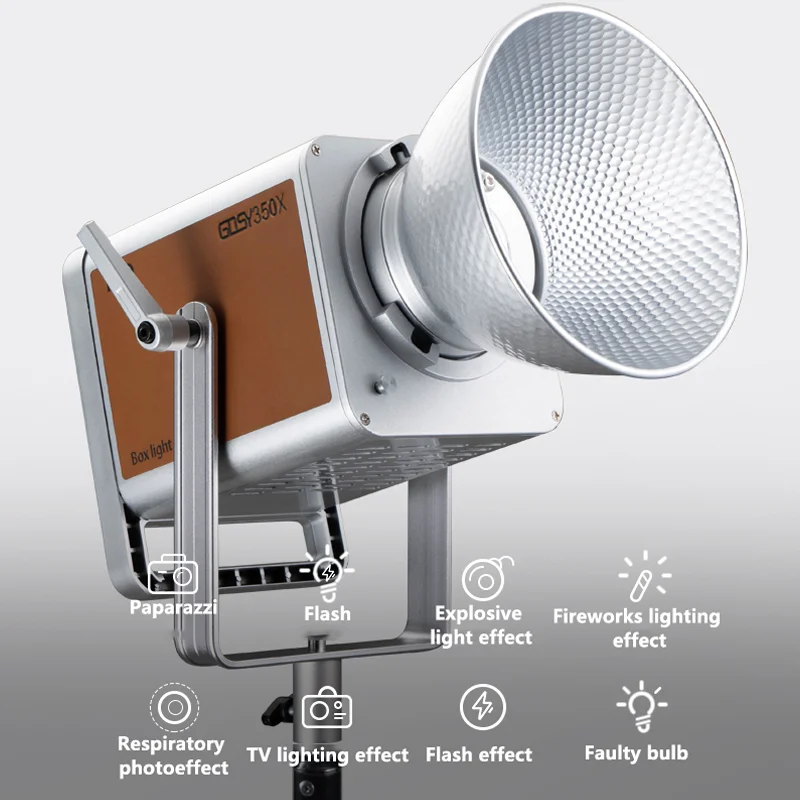This advertisement showcases a high-tech, professional mounted lighting system, likely used in motion pictures or photography. The centerpiece of the image is a squarish metal box mounted on a sturdy U-bracket fixed to a tripod or pole, prominently featuring a reflective funnel, indicating its primary function as a lighting fixture rather than a camera. On the brown side panel of the device, the label "GOSY 350X" is clearly visible. The background transitions from white to gray, highlighting the product's sleek design. At the bottom of the advertisement, a grid of eight simple white graphic elements provides visual details and descriptions: a camera labeled "Paparazzi," a light bulb denoted "Flash," a bomb icon for "Explosive Light Effect," a firework symbol for "Fireworks Lighting Effect," a pattern of concentric circles for "Respiratory Photo Effect," a small television icon for "TV Lighting Effect," a lightning bolt in a circle for "Flash Effect," and a light bulb with rays extending outward for "Faulty Bulb." This detailed layout suggests the versatile lighting capabilities of the GOSY 350X, making it an essential tool for any advanced photographic or filmmaking setup.